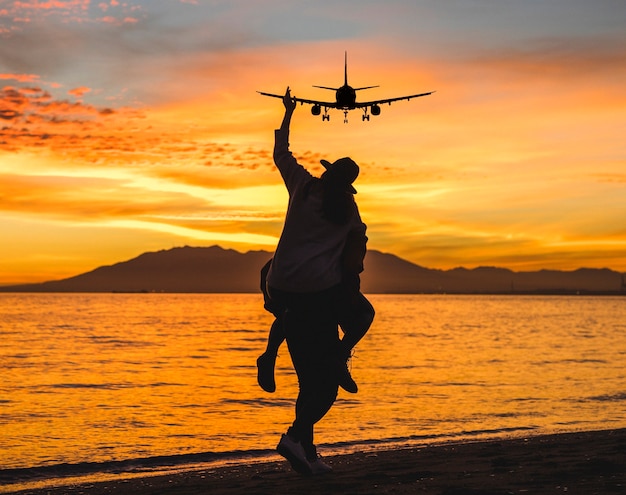At sunset, a captivating photograph captures the scene by a tranquil body of water, possibly a lake or ocean. The sky is ablaze with bright orange and deep yellow hues, blending into pinks as dusk settles in. Silhouetted against this vivid backdrop is an airplane, positioned centrally in the upper part of the sky, either flying away or towards some distant airport.

On the shoreline beneath the airplane, two figures can be seen. One person, possibly a young woman, is perched on the back of another person, perhaps a young man. This man, wearing a hat, holds her steady as her legs dangle to his side. Her arm is extended upwards with an almost magical alignment, making it appear as if she is touching the wing of the airplane high above.

Their silhouettes stand against the glistening orange-tinted water, with a majestic series of mountains faintly visible on the horizon. The photograph, taken from the foreground on the near side of the water, beautifully captures this moment of playful interaction and serene natural beauty, as the duo appears to be waving goodbye to the plane amidst the enchanting colors of sunset.